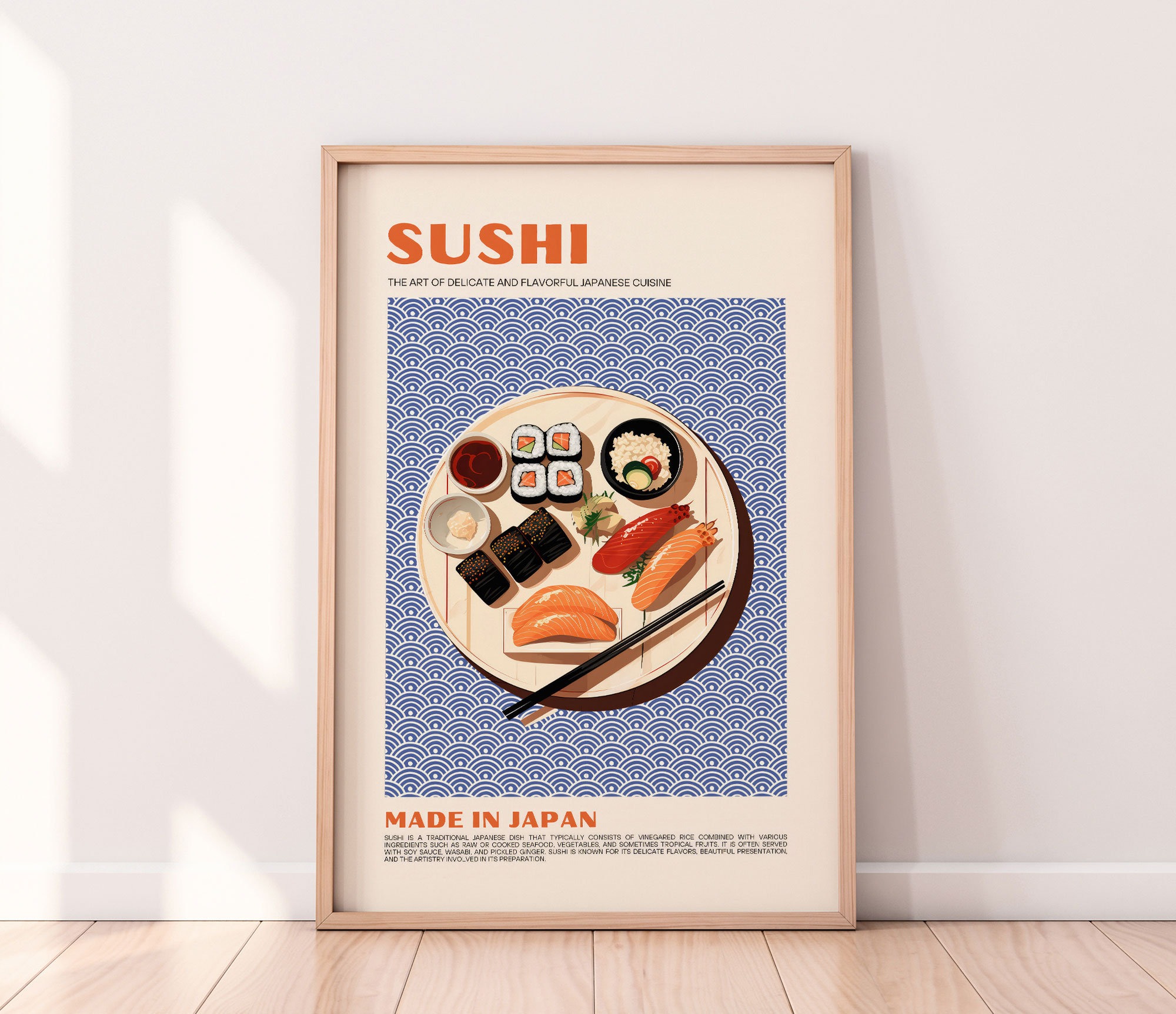The image showcases a vertically-oriented art piece with a light wooden frame, standing on a pristine beige wooden floor, adjacent to a white wall with trim. The focal point of the framed poster is a beautifully arranged platter of sushi, captured from a top-down perspective. Across the top of the poster, bold orange letters spell "Sushi," followed by the subtitle "The Art of Delicate and Flavorful Japanese Cuisine" in smaller black lettering. The sushi plate rests on a blue mat with scalloped patterns, adding a touch of elegance.

The plate itself is adorned with an assortment of sushi, including four cut rolls, approximately four nigiri rolls, a small bowl of soy sauce, a bowl of ginger, and another with a tan material, possibly rice. Additionally, there are black pieces, enhancing the plate's variety. A single chopstick lies diagonally at the lower right corner of the plate. Beneath the detailed depiction of the sushi, the words "Made in Japan" are inscribed in red, with further descriptive text in black at the bottom, elucidating the contents of the plate. This piece exudes an authentic Japanese aesthetic, ideal for a serene restaurant setting.